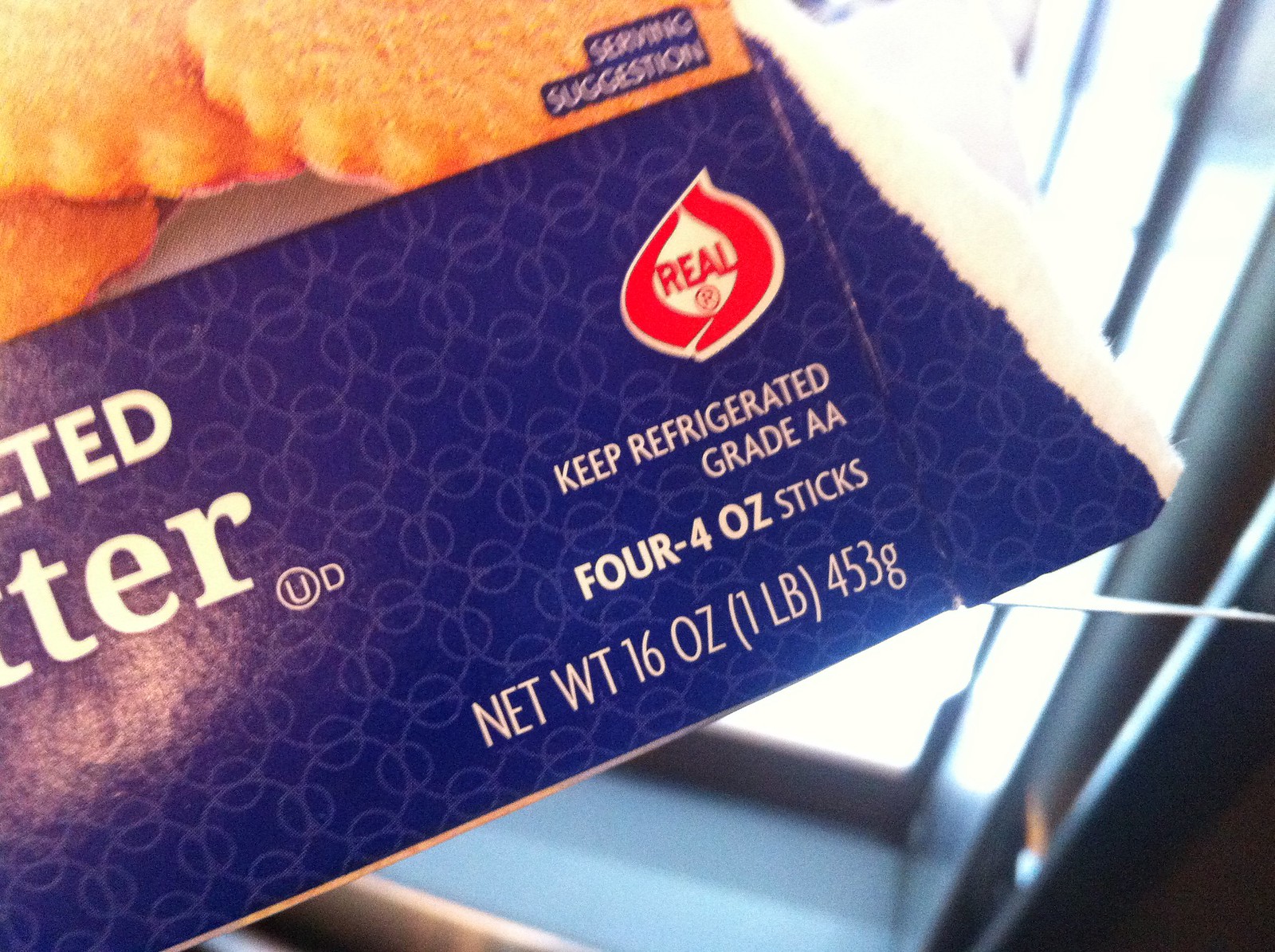This image captures a close-up of the bottom corner of a partially torn package, which seems to be for salted butter. The packaging prominently displays the words "salted butter" and "real," along with a suggestion to "keep refrigerated." The product is described as grade A-A, consisting of four 4-ounce sticks with a total net weight of 16 ounces, or 453 grams. On the blue background section near the torn edge, there's text indicating a "serving suggestion" segment, outlined in blue. The package also features decorative blue circles with smaller circles in between. The text includes fragments in white lettering, with visible portions showing “T-E-D” and “T-E-R." In the background, there's additional context with a window and a silver seal at the bottom.